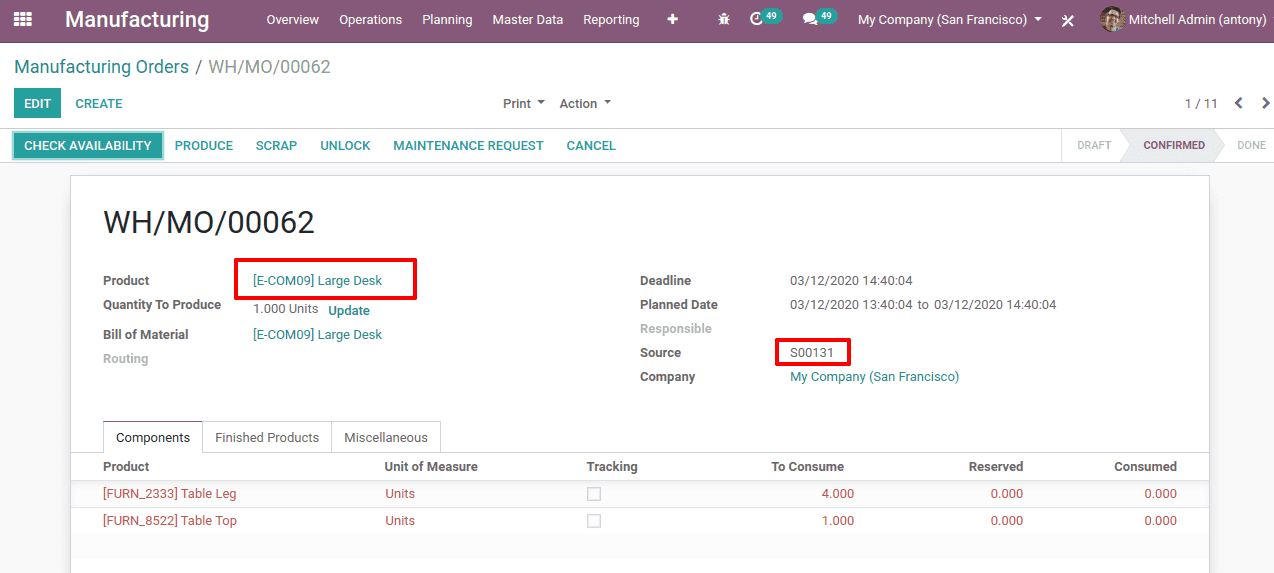This image captures a screenshot of a manufacturing ordering page displayed on a laptop computer screen. Dominating the top portion of the interface, there is a prominent purple horizontal bar featuring the page title "Manufacturing." To the right of this title, a navigation menu presents various options, including "Overview," "Operations," "Planning," "Master Data," "Reporting," and the currently logged-in user, indicated as "Michelle Mitchell (Admin)."

Located below the navigation bar, the main section of the screen provides several functionalities for managing manufacturing orders. Users can enter a part number to check its availability and have options to produce, scrap, unlock, submit a maintenance request, or cancel the order. This interface appears to be part of a specialized computer program designed for use in a manufacturing environment, facilitating efficient ordering and management of parts.